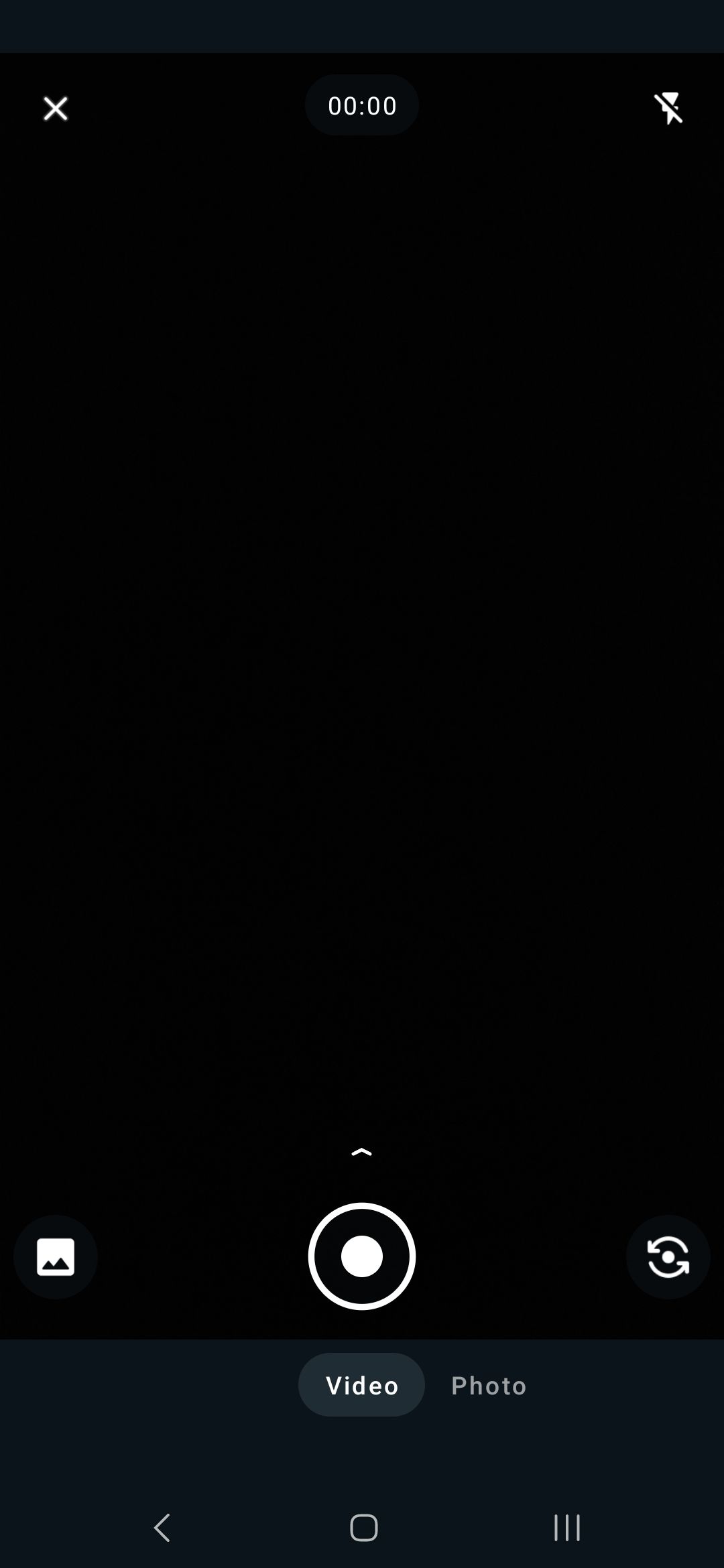A screenshot captures the cell phone camera interface. The top screen features a blue line followed by a sequence of three black boxes. In the top-left black box, a white "X" icon is located, while the middle displays "00:00," and the right side shows a crossed-out flash icon indicating the flash is off. Below these, there's a smaller blue box. The main display area is entirely black, suggesting an obstruction, possibly a thumb, covering the camera lens.

At the bottom interface, there are various icons: a picture gallery icon on the left, a large central button for taking photos, and a button on the right to flip the camera view. Below this central area is the word "Video," highlighted by an oval, adjacent to "Photo." Finally, the bottom-most row includes navigation buttons: a back button on the left, a home button in the center, and an options button (depicted by three horizontal lines) on the right. The overall image suggests the camera app is open but obscured by an object blocking the lens.